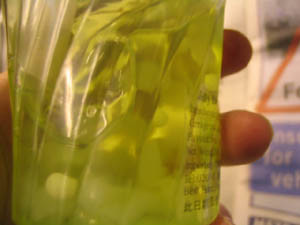This is a close-up photograph of a person's left hand firmly gripping a clear, likely plastic bottle that has a unique spiral shape. The bottle contains a clearish liquid with small green balls suspended inside, giving a slightly sticky appearance. The label on the back of the bottle features a column of black text, although the angle and focus of the photograph make it unreadable. The hand holding the bottle shows visible fingertips, and the background, though blurry, includes a partially visible poster with some lettering and part of an orange triangle. The scene is somewhat ambiguous, leaving the contents of the bottle and the context open to interpretation.